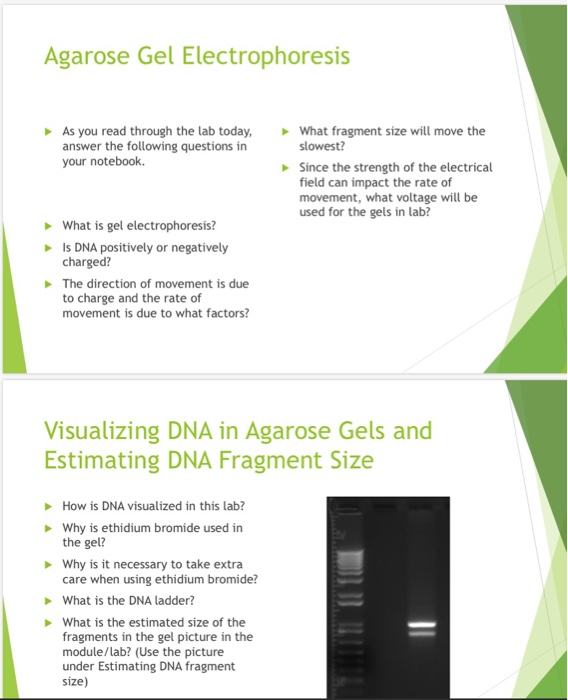The image displays two detailed informational slides focused on DNA analysis using agarose gel electrophoresis. 

**Top Slide (Agarose Gel Electrophoresis)**:
- Title: "Agarose Gel Electrophoresis" in green font.
- Content: Two columns of bullet points, each denoted by green arrows with black text.
- Topics Addressed: Methodology of electrophoresis, potential questions like "How is DNA visualized in this lab?", the usage of ethidium bromide, precautions needed, and explanations about the DNA ladder and fragment sizes.

**Bottom Slide (Visualizing DNA in Agarose Gels and Estimating DNA Fragment Size)**:
- Title: "Visualizing DNA in Agarose Gels and Estimating DNA Fragment Size" in green font.
- Content: Similar bullet points structure, with green arrows and black text for each point.
- Visual Element: Presence of an image to the right, resembling a small black box that looks akin to a refrigerator, potentially illustrating equipment used in the visualization process.
- Additional Details: Left-side column of bullet points discussing fragment size estimation.

**Design Elements**:
- Both slides feature green accents of varying shades on the sides and thin black lines, giving a structured and visually appealing layout suitable for educational purposes, possibly aimed at students or professionals in a symposium or instructional setting.